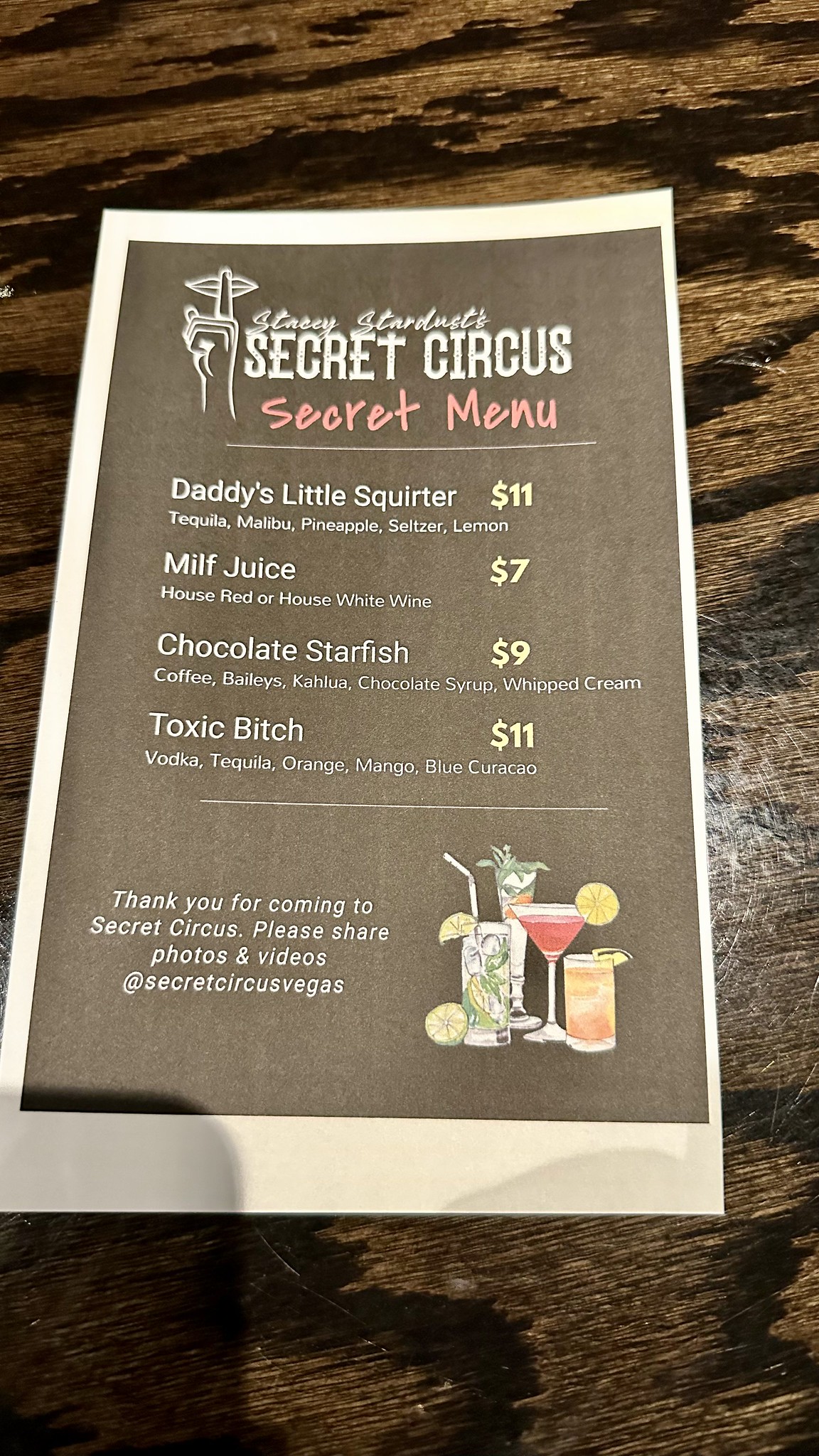A menu sits on a stained pine table, showcasing a sleek design with a white border and a black background. Prominently featured to the left is an image of Stacey Stardust, depicted with a hand over her lips in a shushing gesture. The heading "Stacey Stardust's Secret Menu" is written in striking red letters. The menu items are detailed as follows:

1. **Daddy's Little Squirter ($11)** - Tequila, Malibu, pineapple, seltzer, and lemon. The price is highlighted in yellow.
2. **Milf Juice ($7)** - Choice of house red or house white wine.
3. **Chocolate Starfish ($9)** - Coffee, Baileys, Kahlua, chocolate syrup, and whipped cream.
4. **Toxic Bitch ($11)** - Vodka, tequila, orange, mango, and blue curaçao.

In the bottom right-hand corner, an illustration features an assortment of alcohol glasses. One glass contains an orange drink, another has a raspberry beverage garnished with a lemon slice, and several additional glasses are accompanied by scattered lemon wedges. To the left of these images, in white text, the menu extends an invitation: "Thank you for coming to Secret Circus. Please share photos and videos at Secret Circus Vegas."